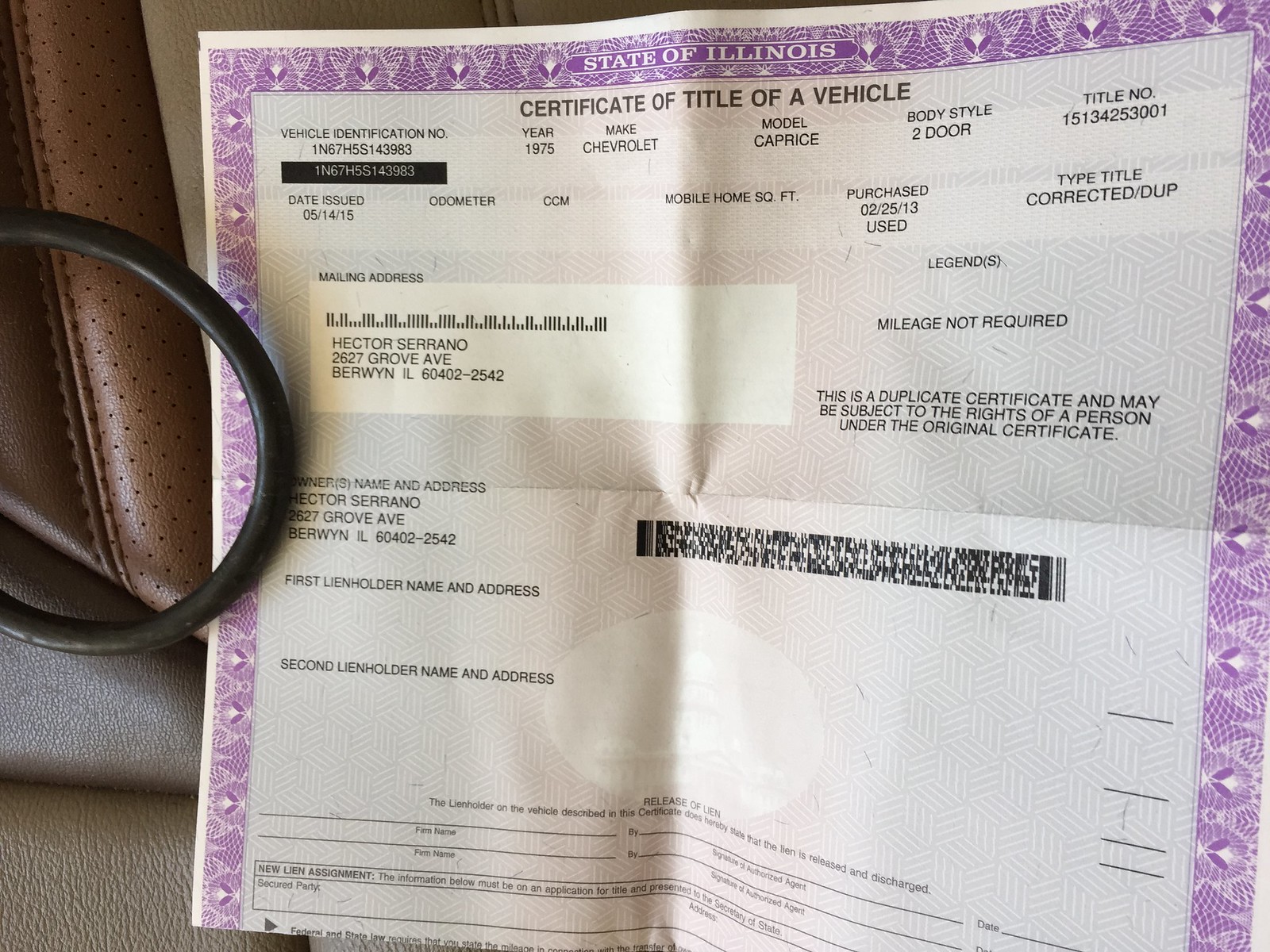This detailed color photograph features an official State of Illinois Certificate of Title for a Vehicle. The document, which appears to be an original title issued on May 14, 2015, for a 1975 Chevrolet Caprice 2-door, has been folded and unfolded and is now lying open on the brown leather seat of a car. The leather seat is partially visible, and a purse strap belonging to a lady is helping to hold the paper in place for the photograph. The title has a distinctive purple border with wavy, leaf-like designs, and at the top, a long rectangular bar with curved edges prominently displays "State of Illinois." The main part of the title has a light purple hue and cube line designs. Key details on the certificate include the vehicle identification number 1N67H5S143983, the title number 15134253001, and the original purchase date of February 25, 2013, for a used vehicle. The owner's mailing address is listed as Hector Serrano, 2627 Grove Avenue, Berwyn, Illinois, 60402-2542. There is also a barcode located in the bottom half of the image. This document is a duplicate certificate, which may be subject to the rights held by a person under the original certificate.